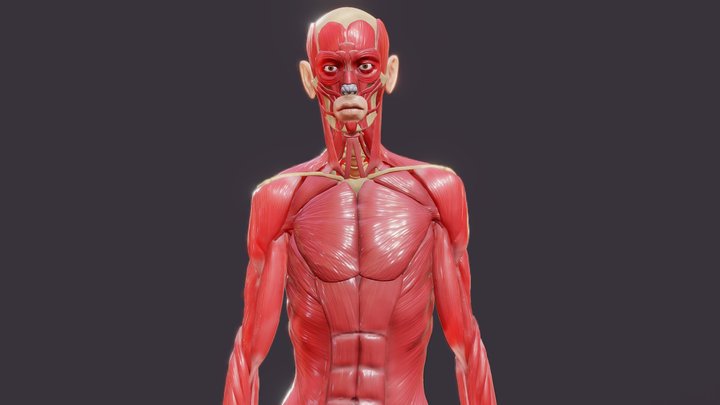This photograph features a mannequin-like model of a human body without skin, set against a dark charcoal or brown background. The mannequin is predominantly red, showcasing detailed muscle tone and tendons. The visible part of the figure spans from the top of the head down to just above the wrists, and includes the pectorals and stomach muscles. Distinctly, the face possesses human-like features with dark eyes, skin-colored ears, and a skin-toned mouth area. Additionally, the top of the head and a triangular pattern stretching from just below the neck to the shoulders display a white person's skin tone.